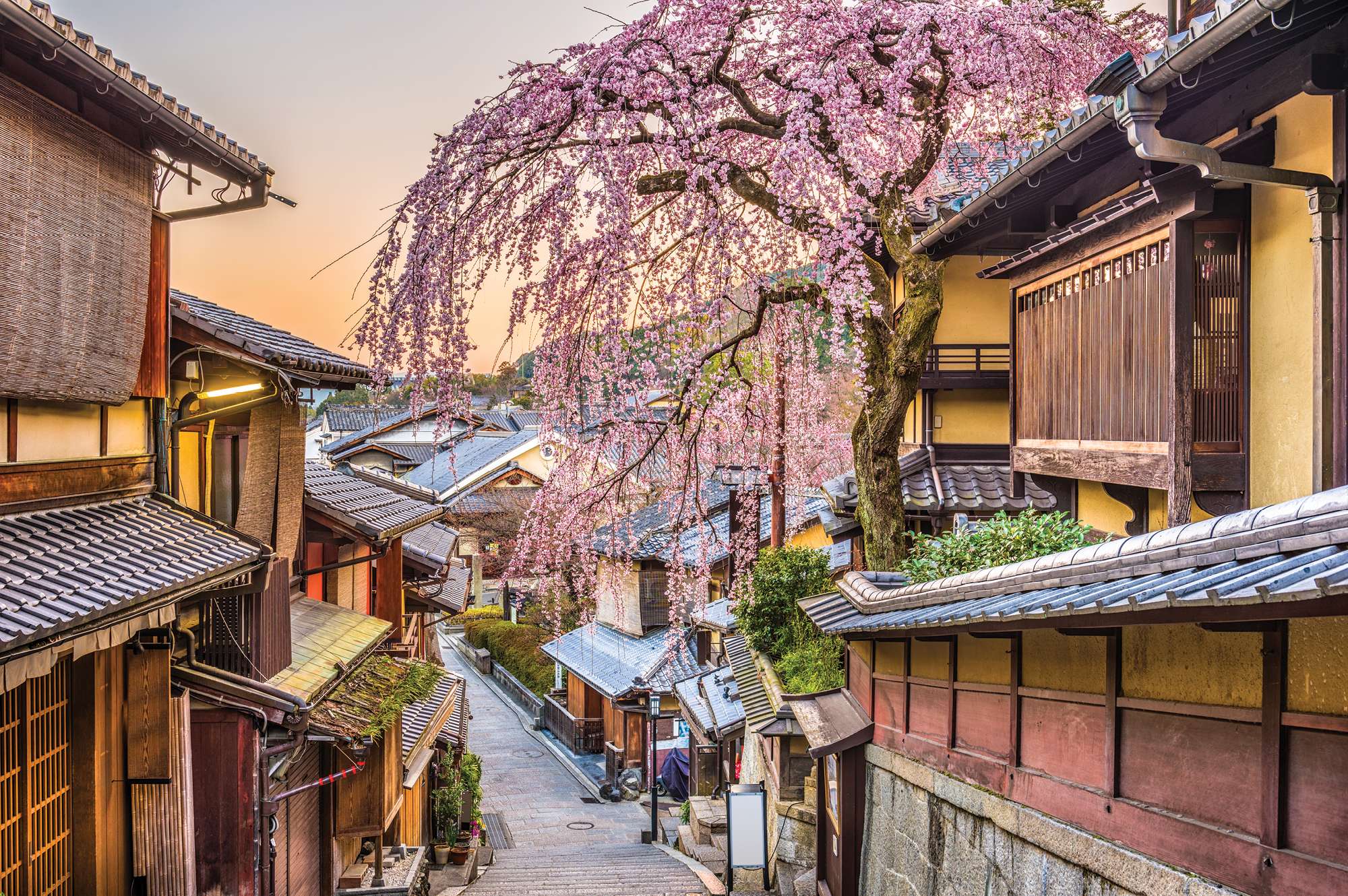This photograph captures the essence of a quaint Japanese town during sunset, with traditional architecture and serene natural elements. At the center bottom of the frame, a narrow grey stone path winds its way up a hill and veers off to the left, bordered by tiered buildings on both sides. These buildings feature shallow metal-topped roofs and traditional wooden structures, including a prominent dark wooden bump-out with vertical slats on the right side. Nestled between the closest buildings on the right is a tall cherry blossom tree, its spindly branches adorned with pink and white petals. 

In the distance on the right side, a sloping green hill peeks out from behind the buildings, complemented by an orangey sky that transitions to blue at the top of the frame, indicating the setting sun. Some lights in the buildings suggest the settling of evening. The street itself is likely too narrow for cars, adding to the charm and historical ambiance of the neighborhood, which appears to have existed for many years. Additional details include hints of green shrubbery and plants along the pathway, a wooden balcony on a yellow house, and several signs in the distance, further enriching the scene.